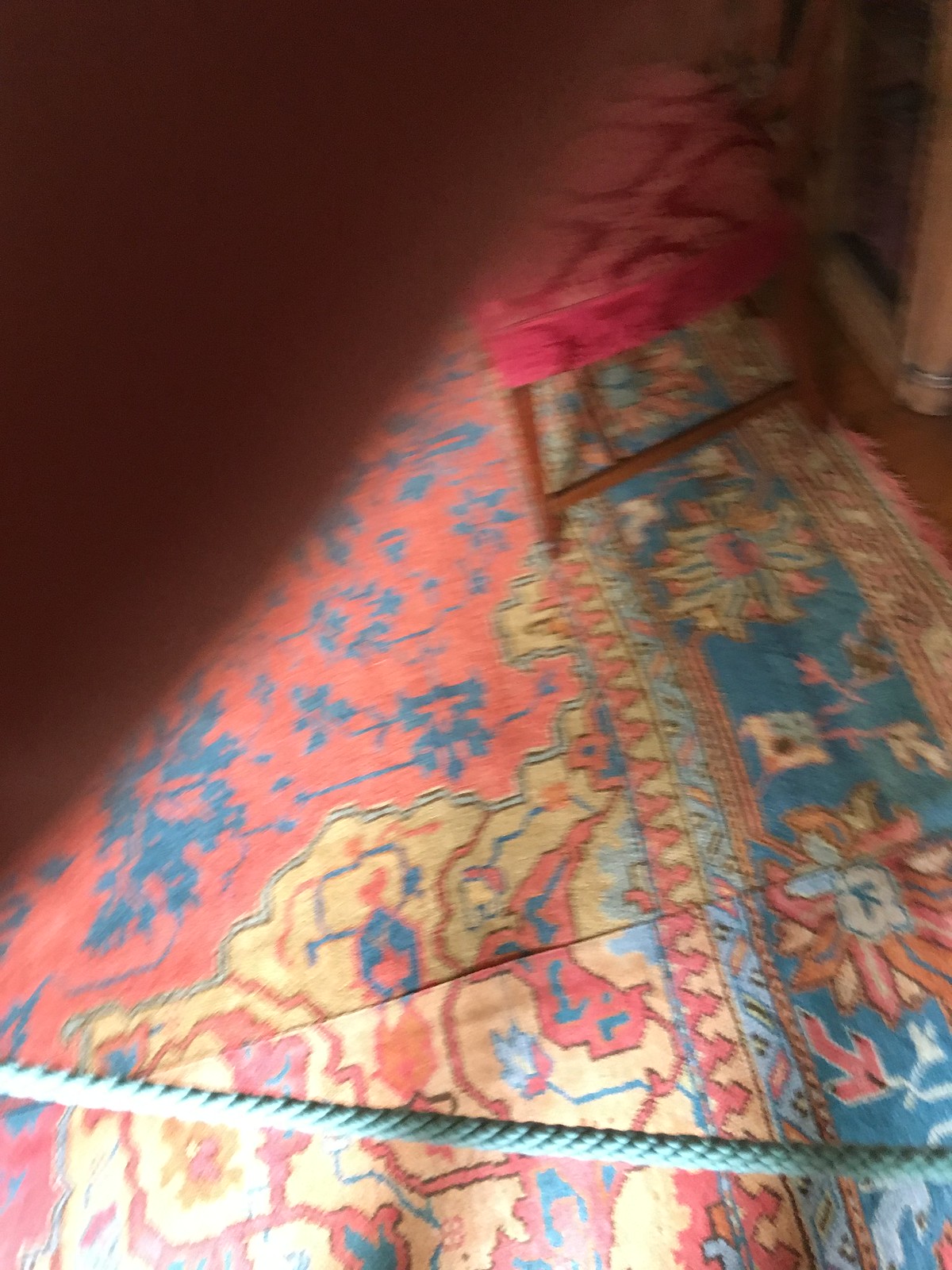The image captures a vertically rectangular frame with a partial obstruction caused by a finger covering the lens. This obstruction starts just below the center on the left side and extends diagonally up to just right of center at the top, making the entire left side of the image blurred. The visible portion of the scene reveals a detailed look at a domestic setting. 

In the upper-right quadrant of the image, there is a dark brown wooden chair with a red velour-textured seat, suggesting a vintage or classic style. The seat is placed on a large, ornate carpet adorned with floral decorations in shades of orange, blue, and tan.

Towards the bottom of the frame, spanning from left to right at a slight downward angle, there is a blue rope, possibly part of some household item or furnishing. The remainder of the scene downward appears to be a view of a cushioned area on the carpet, contributing to the cozy and intricate ambiance of the setting.